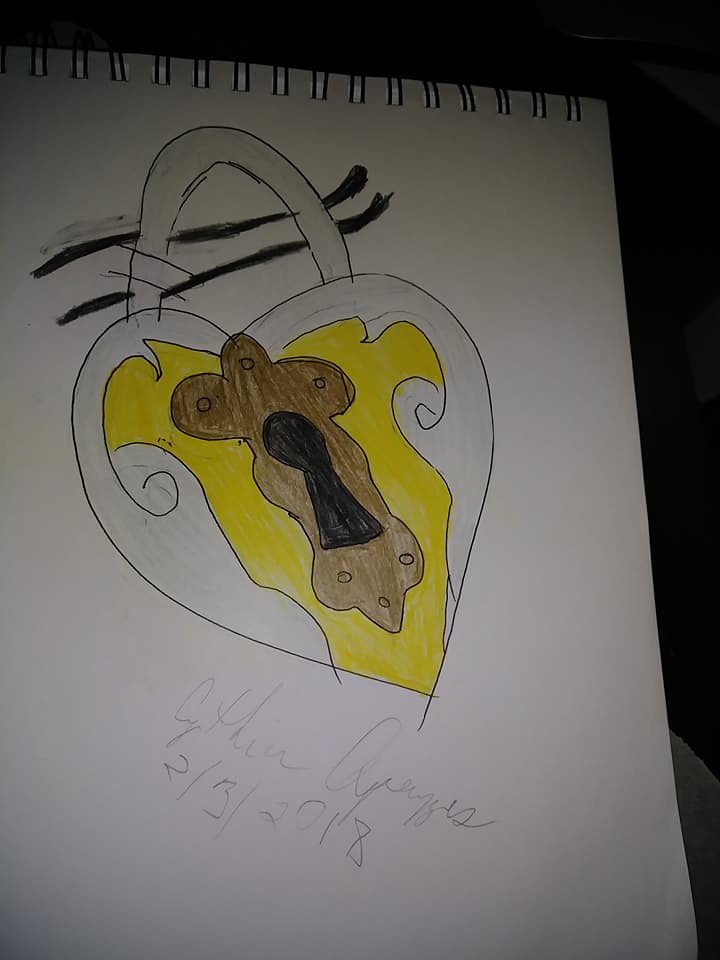This photograph captures a piece of artwork hand-drawn in a spiral notebook, with the image taken using a flash against a dark background, emphasizing the intricate details of the drawing. Central to the artwork is a finely detailed heart-shaped locket, reminiscent of those used on diaries or seen adorning the famous lock bridge in Paris. The locket features a small keyhole set into a plate, drawn in black and surrounded by a golden-brown area mimicking the look of an ornate metal plate. The body of the locket is primarily yellow with delicate swirly designs, while the edges remain white, creating a striking contrast. The drawing appears to be executed with a combination of pen, marker, and possibly crayon, with wavy lines in the background suggesting the locket is hanging on a fence or another type of support. At the bottom of the page, there is a light, pencil-rendered signature and a date, possibly reading 2/3/2018, though the name of the artist is difficult to decipher.